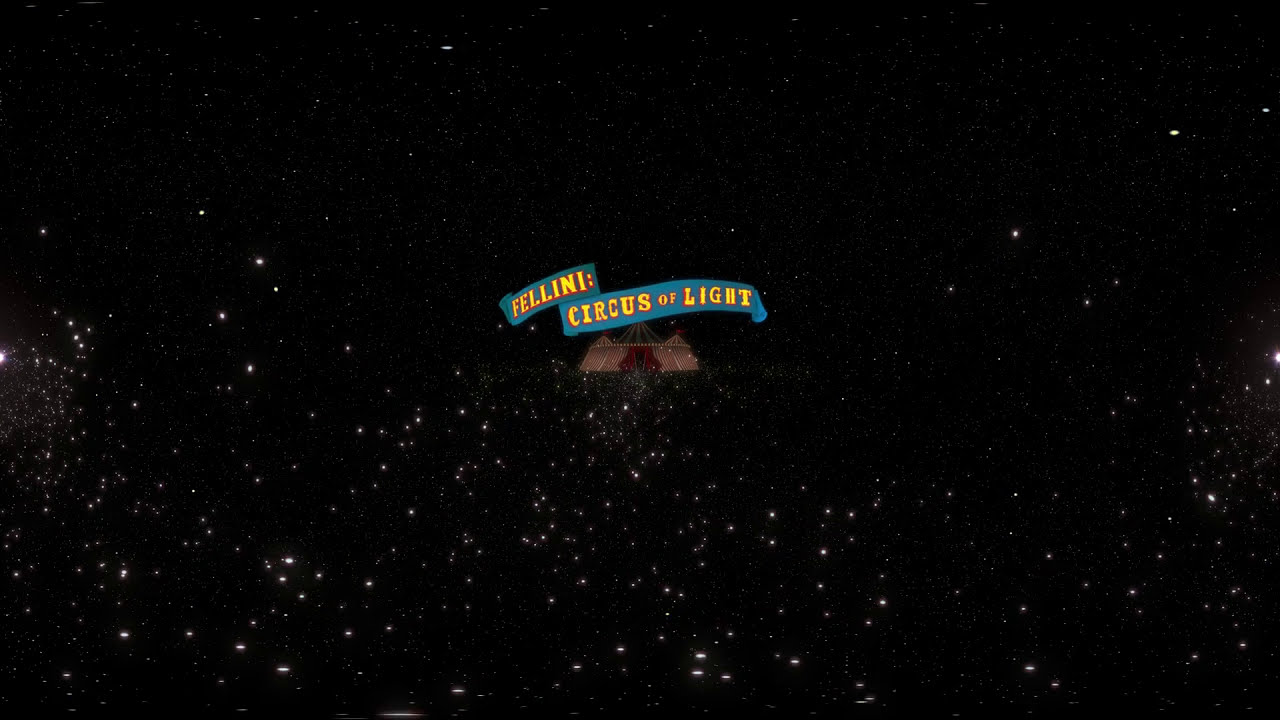The image depicts a vast, black night sky dotted with an infinite number of white stars, with the brightest stars concentrated mainly on the bottom half and smaller, fainter stars scattered across the top half. Dominating the center of this cosmic background is a vibrant blue banner with yellow text that reads "Fellini: Circus of Light." Below the banner, a striking red and white striped carnival tent with three large peaks is prominently featured, complete with red flags adorning the tops of the peaks and a red entrance at the center. The vivid colors and intricate details of the tent stand out against the dark, starry expanse, creating a mesmerizing, whimsical focal point in the image.